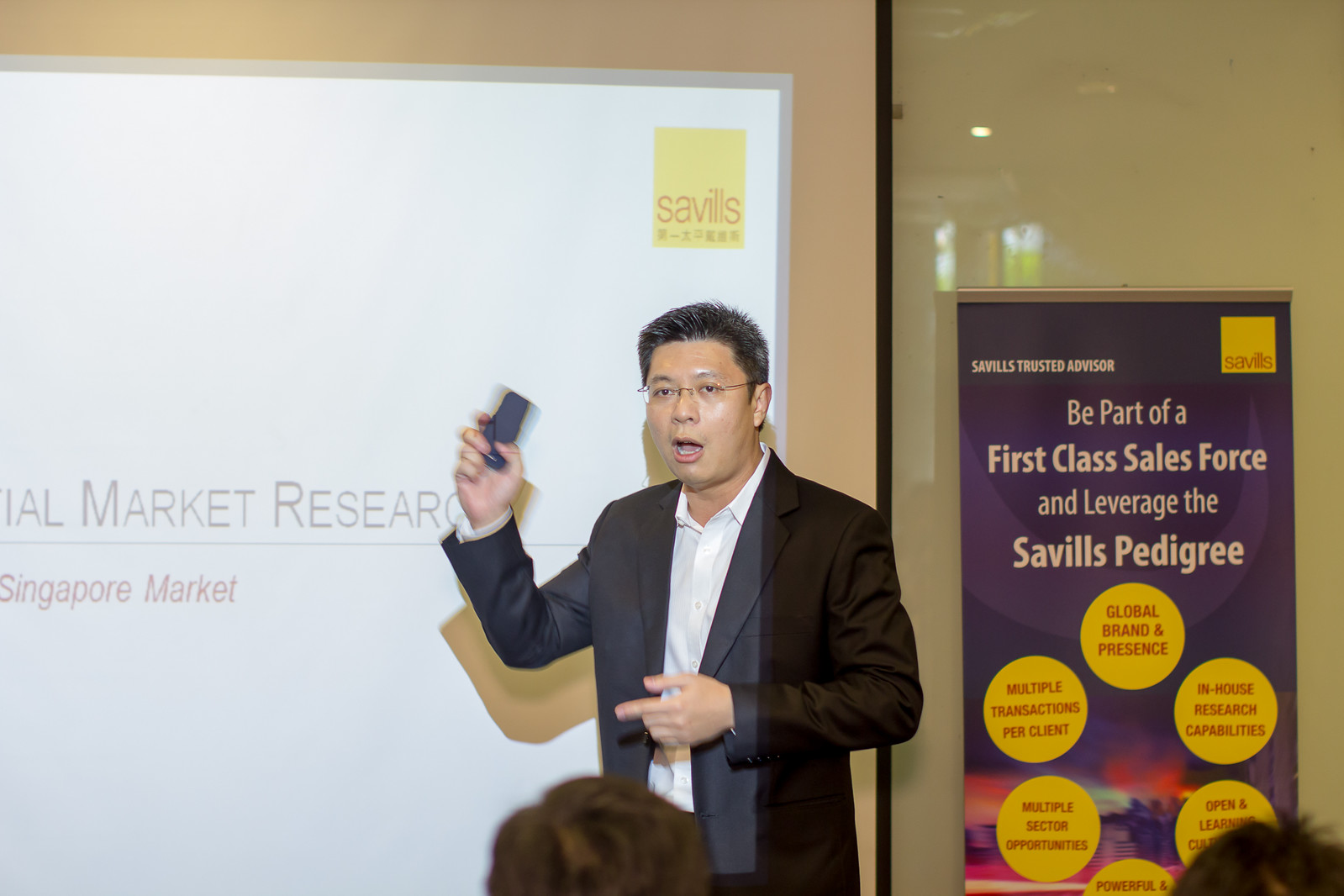The photograph captures an Asian gentleman in mid-speech at a conference, wearing a dark business suit and white shirt, with glasses. He holds a projector clicker in his right hand, which he points towards a projection behind him onto a tan wall. The partial projection includes phrases like "IAL Market Research" and "Singapore market". To his left hangs a sign reading "Savillis Trusted Advisor. Be part of a first-class sales force and leverage the Savillis pedigree," accompanied by six yellow bubbles outlining benefits such as global brand presence, multiple transactions per client, multiple sector opportunities, in-house research capabilities, open and learning culture, and a partially visible phrase starting with "powerful." Behind him is a floor-to-ceiling window, adding to the professional ambiance of the scene.